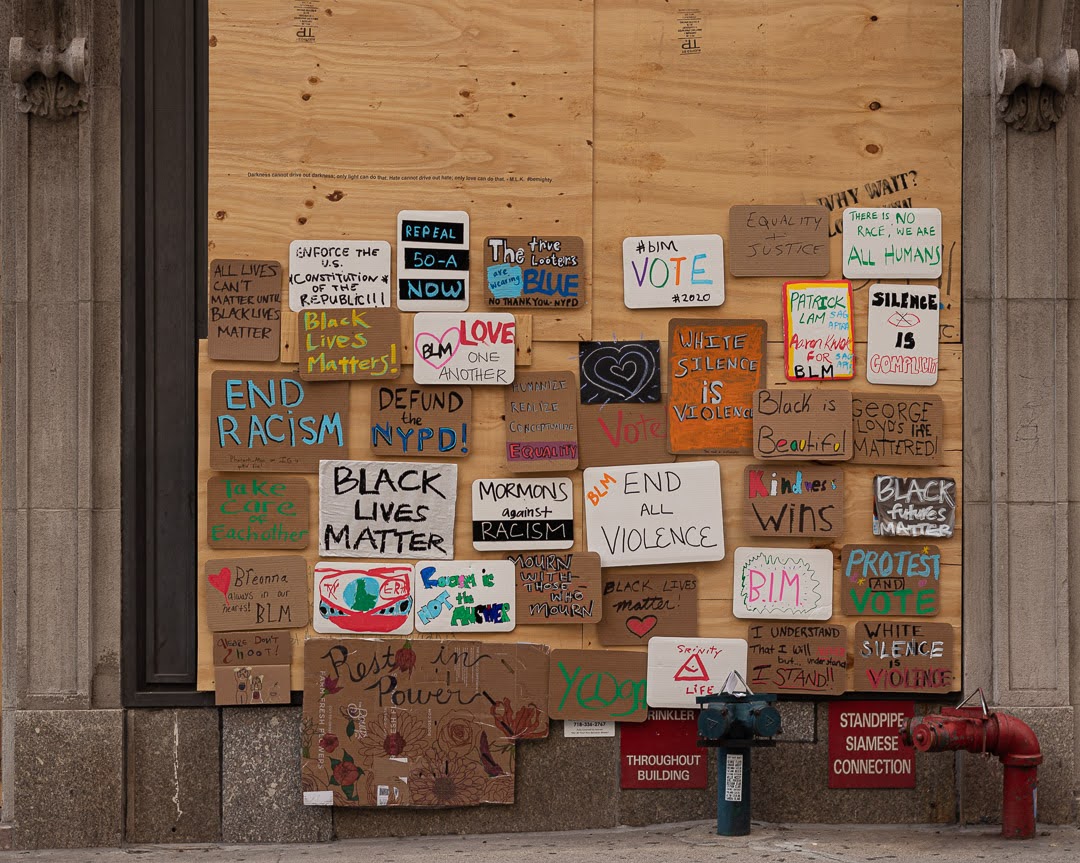The image shows a rectangular photograph of a gray concrete wall in an outdoor setting. The ground is also concrete, and the building itself appears to be constructed from the same material. Covering parts of the wall are several plywood boards, nailed securely in place. On the bottom right-hand side of the image, two distinct pipes or connectors can be observed: one red, slightly resembling a fire hydrant, labeled with a sign that reads "Standpipe Siamese Connection," and a blue one of a different shape, accompanied by a red sign stating "Sprinkler Throughout Building."

Attached to the plywood boards are numerous handmade signs, mostly crafted from cardboard and displaying a variety of messages. These signs serve as both a tribute and a protest, with slogans including "End Racism," "Defund the NYPD," "Black Lives Matter," "End All Violence," "Protest and Vote," "Kindness Wins," "White Silence is Violence," "Vote," "Love One Another," and "Rest in Power." There is also a striking black rectangle with a white heart in the center. Scrawled across the different boards are an array of colors—blue, black, white, red, green, and orange—adding vibrancy to the wall.

This plywood-covered wall, possibly boarding up the windows of a building that seems to be shut down, has transformed into a poignant tribute wall dedicated to Black Lives Matter, showcasing the community's messages of hope, solidarity, and demand for justice.